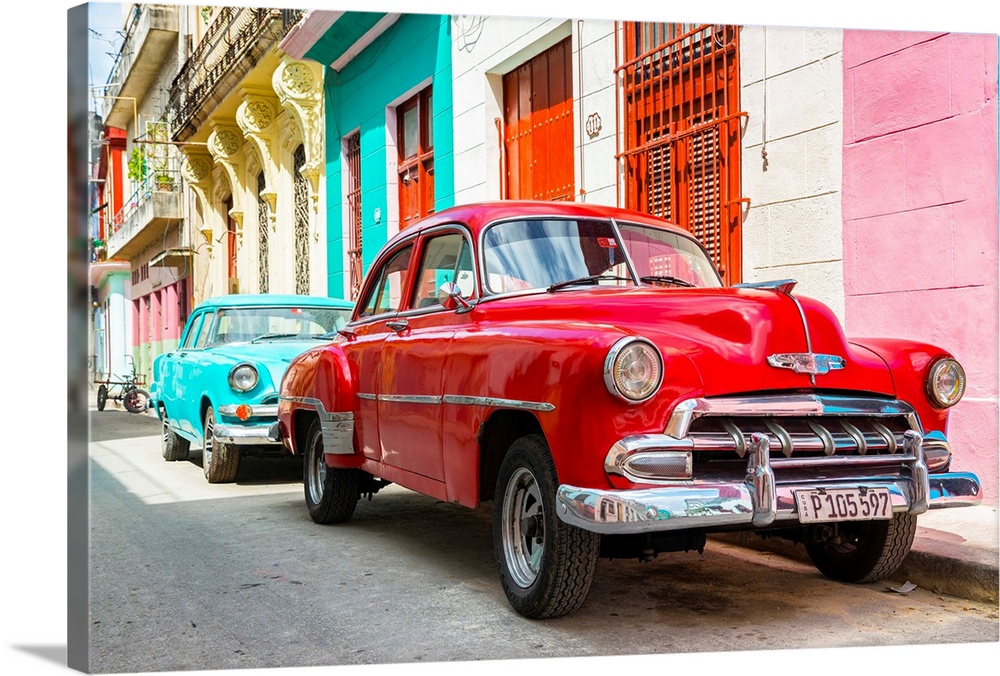This photograph, set in Cuba, showcases two vintage Chevrolet Bel Airs parked on the side of a vibrant, colorful street in a village. The street runs diagonally from the lower right-hand corner to about midway on the left side of the image. The car in the front is a gleaming cherry red Chevy with the license plate reading P105597, adorned with shiny chrome and silver accents. Behind it is a cerulean or teal blue Chevy, equally well-preserved and reminiscent of the classic automobiles for which Cuba is famous. The cars are separated from the brightly painted buildings by a narrow sidewalk. The buildings, constructed from large stone bricks, display a lively palette including shades of pink, white with red doors, a teal building matching the color of the second car, and possibly yellow. They feature ornate wrought iron railings on their upper balconies. The image captures the cars up close, emphasizing their vintage charm against the backdrop of a sunny day highlighting the rich hues and architectural details of the Cuban street.